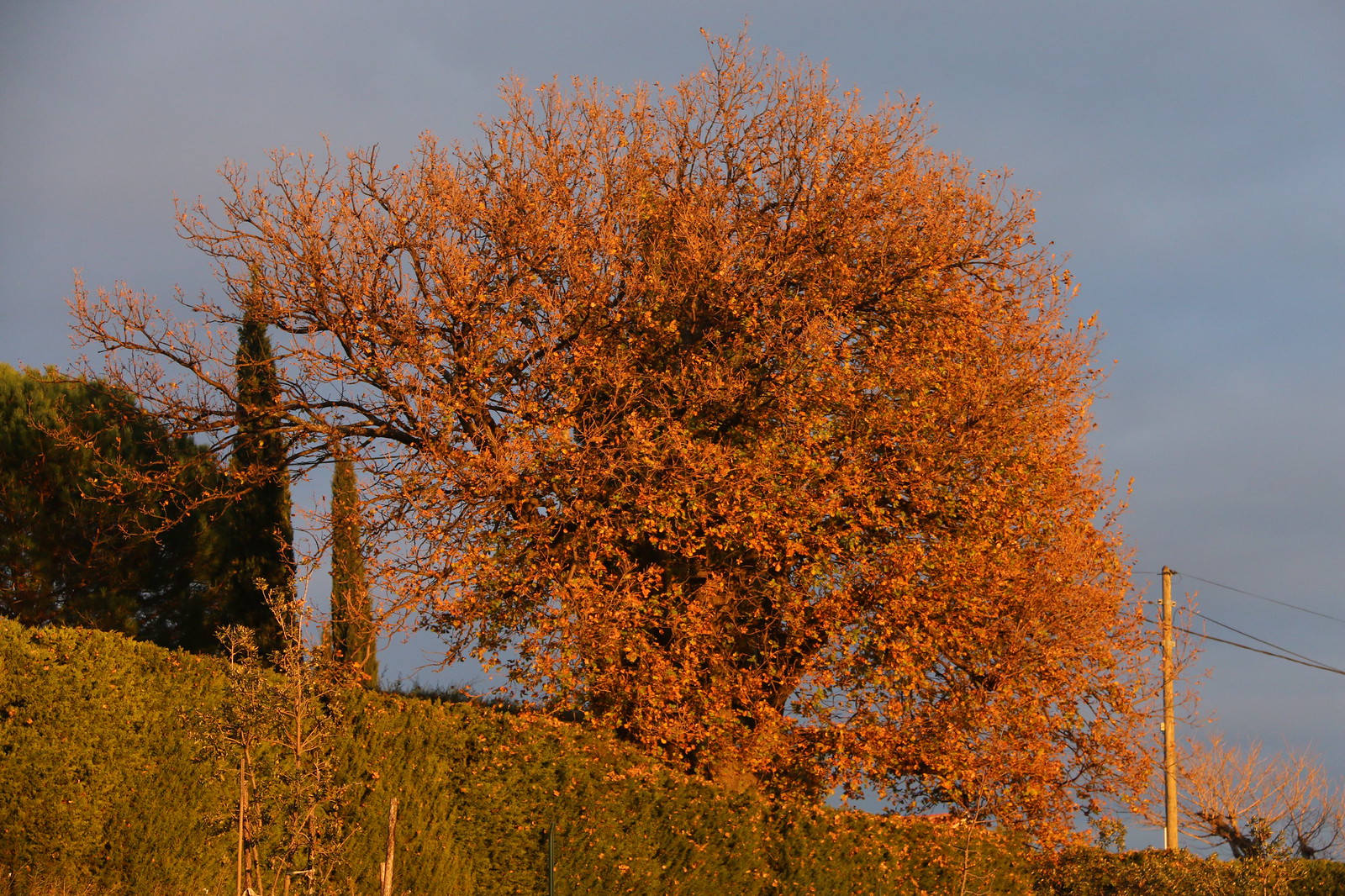In the center of the image stands a large, evidently aging tree that serves as the main focal point. The tree, likely in the fall season, showcases an array of leaves in shades of brown, beige, orange, and a dark golden hue, evident of the season’s characteristic transformations. Several branches are devoid of leaves, emphasizing its transitional state. The base of the tree is surrounded by green, mossy grass atop a small hill, and a bush beneath it is scattered with fallen leaves. 

To the left in the background, a line of green, evergreen trees and possibly garden pine trees provide a contrasting backdrop. On the right side, an electrical power pole with black or brown lines crossing behind the scene adds a touch of human infrastructure to the natural setting. The sky appears overcast or slightly colored by the setting sun, contributing a serene lighting that bathes the entire landscape. The meticulous detailing of the foliage and surroundings, in conjunction with the midday look, suggests that this could be a digital art piece rather than a photograph.